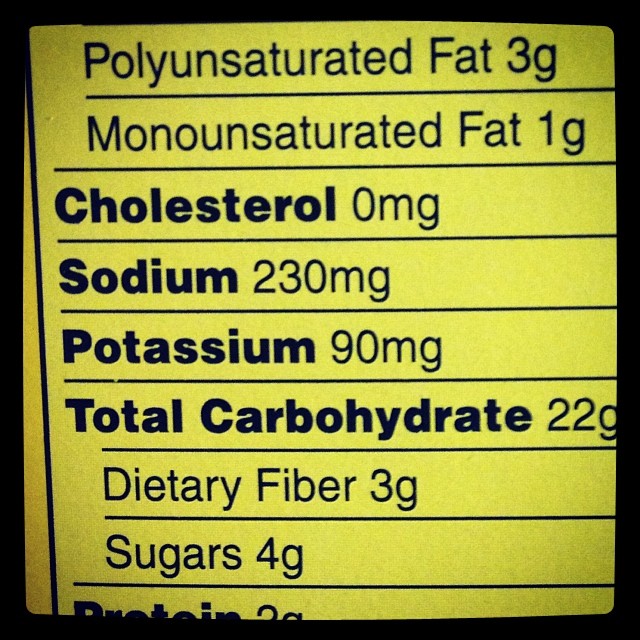Nutritional Information Panel:

A close-up image captures a segment of a nutritional facts label framed by a yellow-lined border. The visible portion lists the following details:
- Polyunsaturated Fat: 3 grams
- Monounsaturated Fat: 1 gram
- Cholesterol: 0 milligrams (in bold font)
- Sodium: 230 milligrams (in bold font)
- Potassium: 90 milligrams (in bold font)
- Total Carbohydrates: 22 grams (in bold font)
- Dietary Fiber: 3 grams
- Sugars: 4 grams
- Protein: The top part of the word "Protein" is visible, along with the partial figure "2 grams."